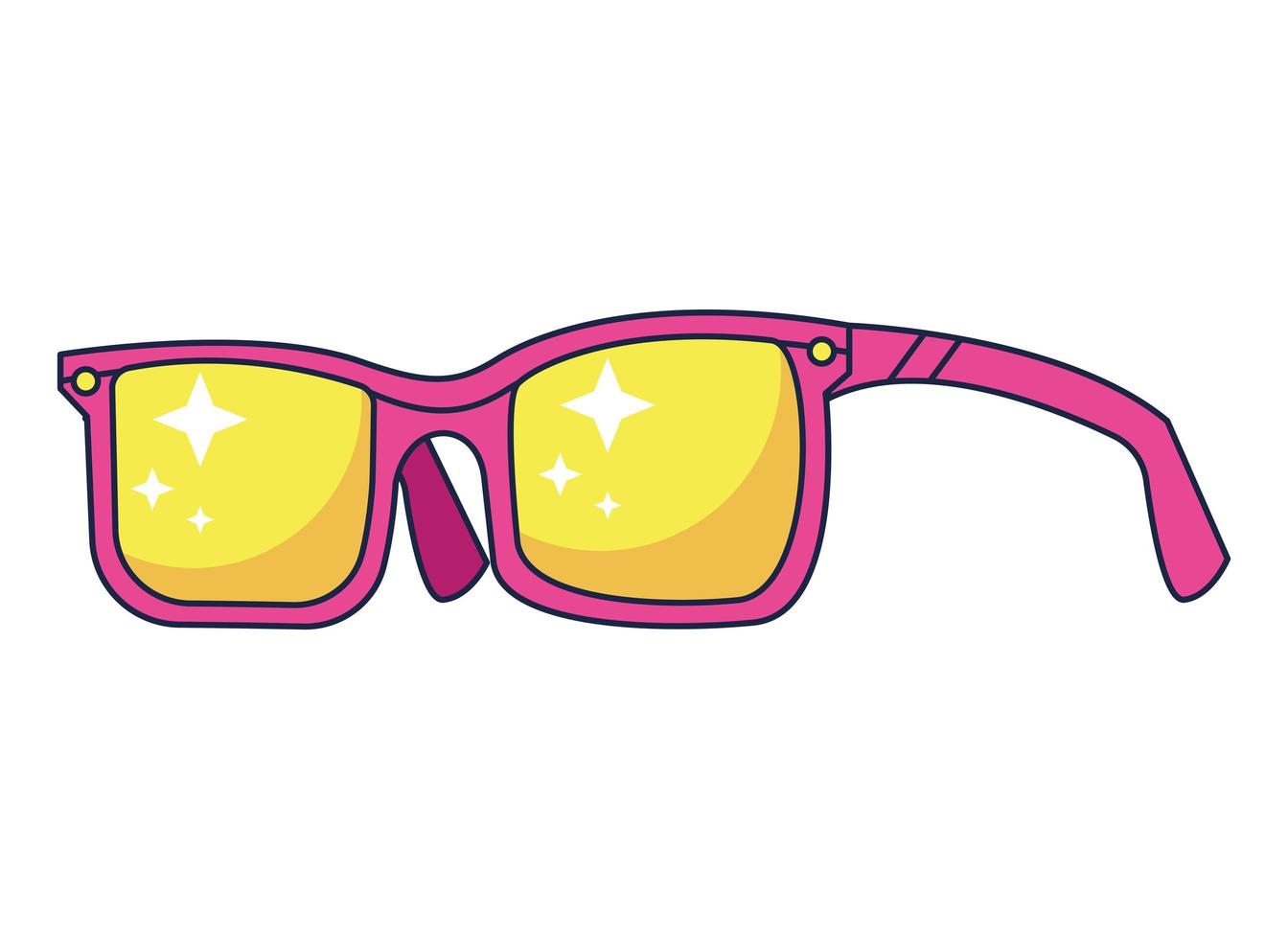This vibrant cartoonish illustration depicts a pair of bright pink sunglasses with a playful, exaggerated comic book style. The sunglasses feature golden yellow lenses, each adorned with three white, four-pointed star shapes reminiscent of the Bethlehem star, creating a magical, twinkly effect. The frames slightly dip in the middle and are decorated with two small yellow dots above the lenses, adding a whimsical touch. These sunglasses are tilted at an angle, with one ear piece visible while the other is tucked behind. The overall color scheme is eye-catching, with bright pink and yellow hues drawing immediate attention. The lenses' shading gives the impression of looking into the bright sun or sparkling stars, enhancing the lively and joyful appearance of the image.